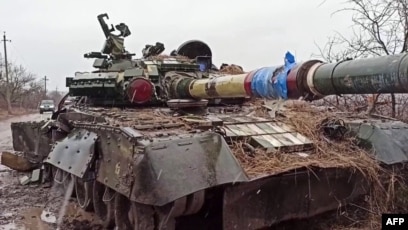An abandoned, battle-worn army tank, with a dark gray and black, shiny body, sits in disrepair on the roadside under a somber, cloudy sky. The tank is covered in a mix of dead leaves, branches, and pine needles, giving it a neglected, forgotten look. Its large front cannon, wrapped in blue tape, points outward, while numerous dents and malfunctioning side panels emphasize its rough history. Parts of the tank, including latches and side panels, are visibly open or falling apart. A legged sign leans against its near side, and debris is scattered across its top. Nearby, a car with headlights on drives along the adjacent road, bordered by trees, including a bare deciduous tree on one side, highlighting the wilderness setting.